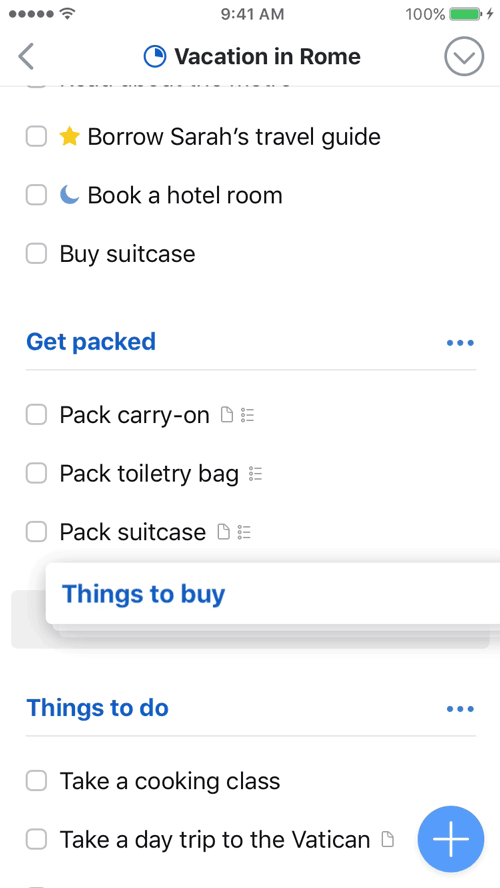The image is a screenshot of a smartphone display taken at 9:41 a.m., showing a fully charged battery indicated at 100% and a full signal strength. At the top of the screen, there's a back arrow icon. The main heading "Vacation in Rome" is accompanied by a drop-down arrow for further details. Below this heading, there is a to-do list with various items:

1. "Borrow Sarah's travel guide" highlighted with a yellow star icon.
2. "Book a hotel room" marked with a moon icon.
3. "Buy a suitcase."

Each item has a checkbox next to it for tracking completion. The next section is "Get Packed," which has a series of sub-items:

- "Pack carry-on," accompanied by a file icon and three horizontal lines.
- "Pack toiletry bag," also with a file icon and three horizontal lines.
- "Pack a suitcase," similarly depicted with a file icon and three horizontal lines.

Each of these sub-items also has a checkbox for completion tracking. The following section is "Things to Do," featuring the items:

- "Take a cooking class."
- "Take a day trip to the Vatican," including a file and picture icon.

At the bottom of the list, there is a prominent blue circle with a plus sign, likely used for adding new tasks or notes.